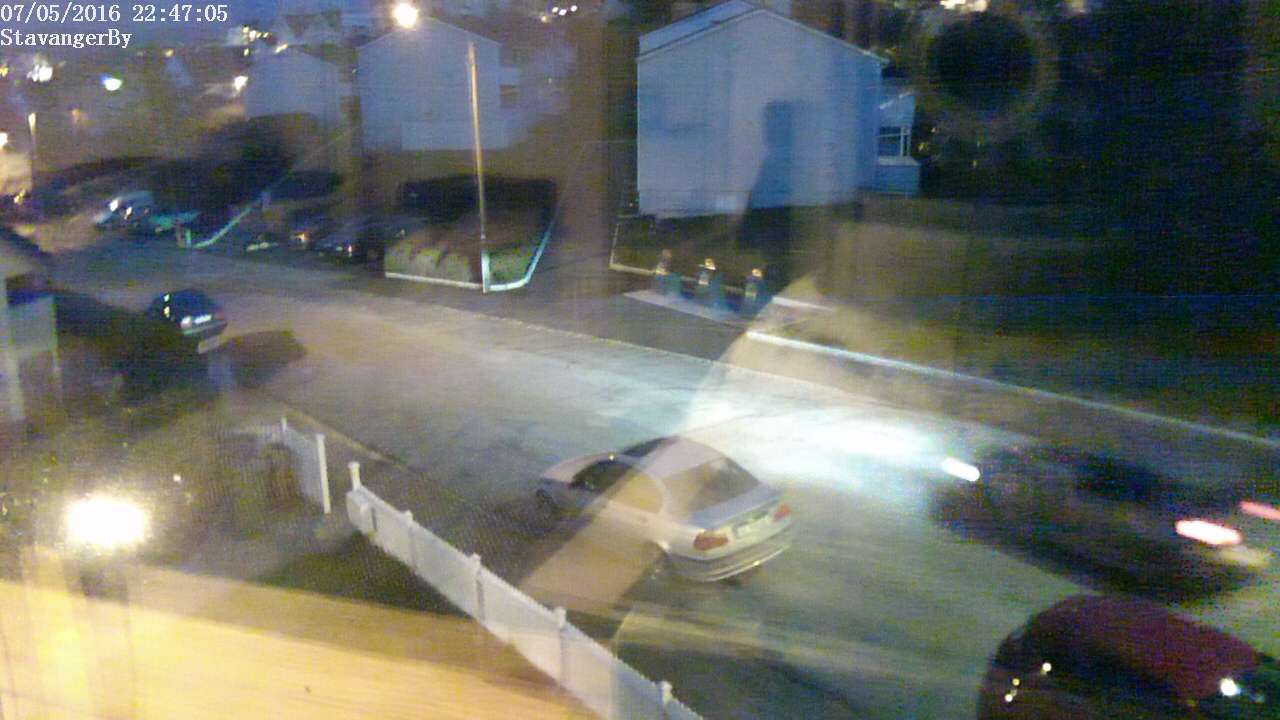This nighttime photograph captures a two-lane neighborhood road, featuring a slight overexposure and a hint of blurriness. The scene is timestamped "07-05-2016" at 22:47:05 (military time). On the right side, there is a parking lot with an adjacent driveway leading to it, flanked by a series of two- to three-story apartment buildings. The road hosts three to four vehicles, primarily sedans. Specifically, a red or burgundy sedan is visible at the bottom right, a silver sedan is near the center, and a gray-green sedan is positioned further ahead. On the left side of the road, a white picket fence runs parallel to the street, accompanied by a driveway and front yard lights, adding a touch of suburban charm to the scene.